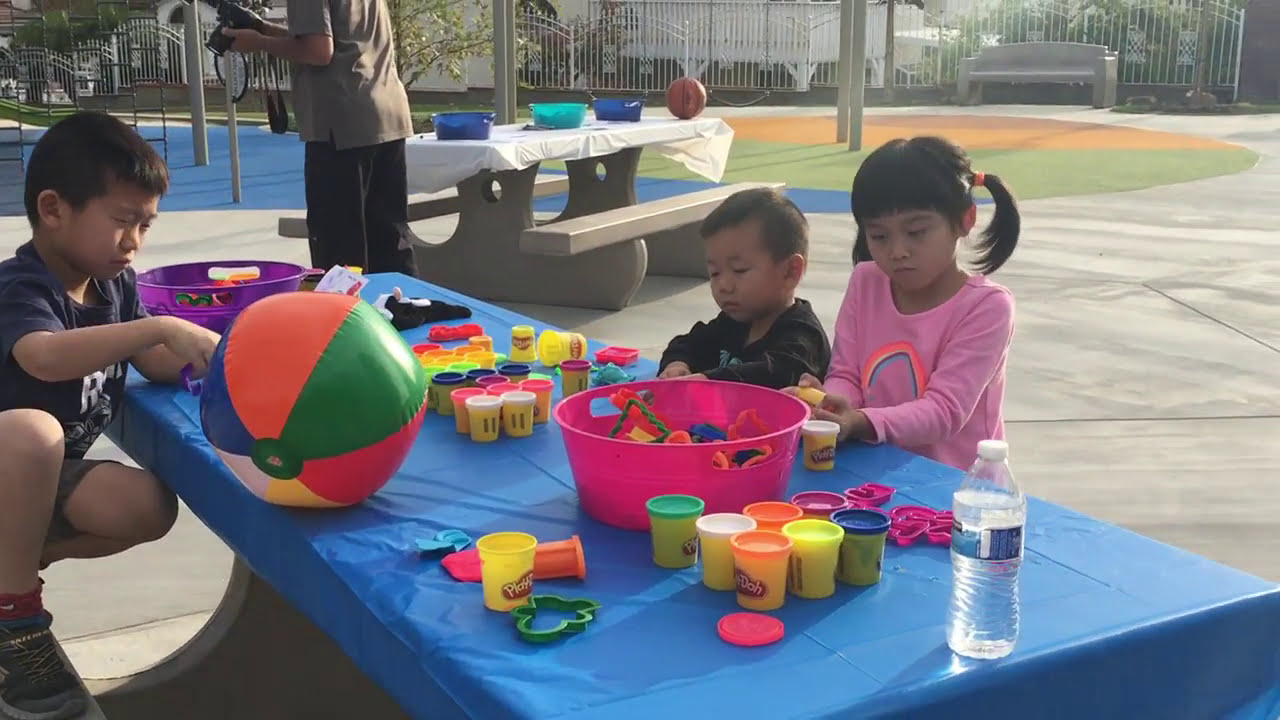In this vibrant outdoor photo taken during the day at a park, three Asian children are the focal point as they engage enthusiastically with an array of toys and colorful Play-Doh at a picnic table covered in a blue tablecloth. Centered in the image, a girl with two pigtails stands out in her pink long-sleeved shirt adorned with a rainbow, directing her activities with the Play-Doh. Beside her on the right stands a smaller boy dressed in a black shirt, equally engrossed in the playful chaos of the table. Across from them, another boy perches on top of the picnic bench, his attention fixed on a brightly colored beach ball with segments of green, orange, blue, yellow, and white. Around them, the table is laden with more jars and containers of Play-Doh, a red tub, a purple bowl, a large pink bowl, and a half-full bottle of water. The park in the background features more picnic tables with bowls scattered on them, a playground area with distinctive orange and green markings on the pavement, and a few trees to the left. The scene captures a lively moment of play and camaraderie amongst the children in a spacious and colorful park setting.